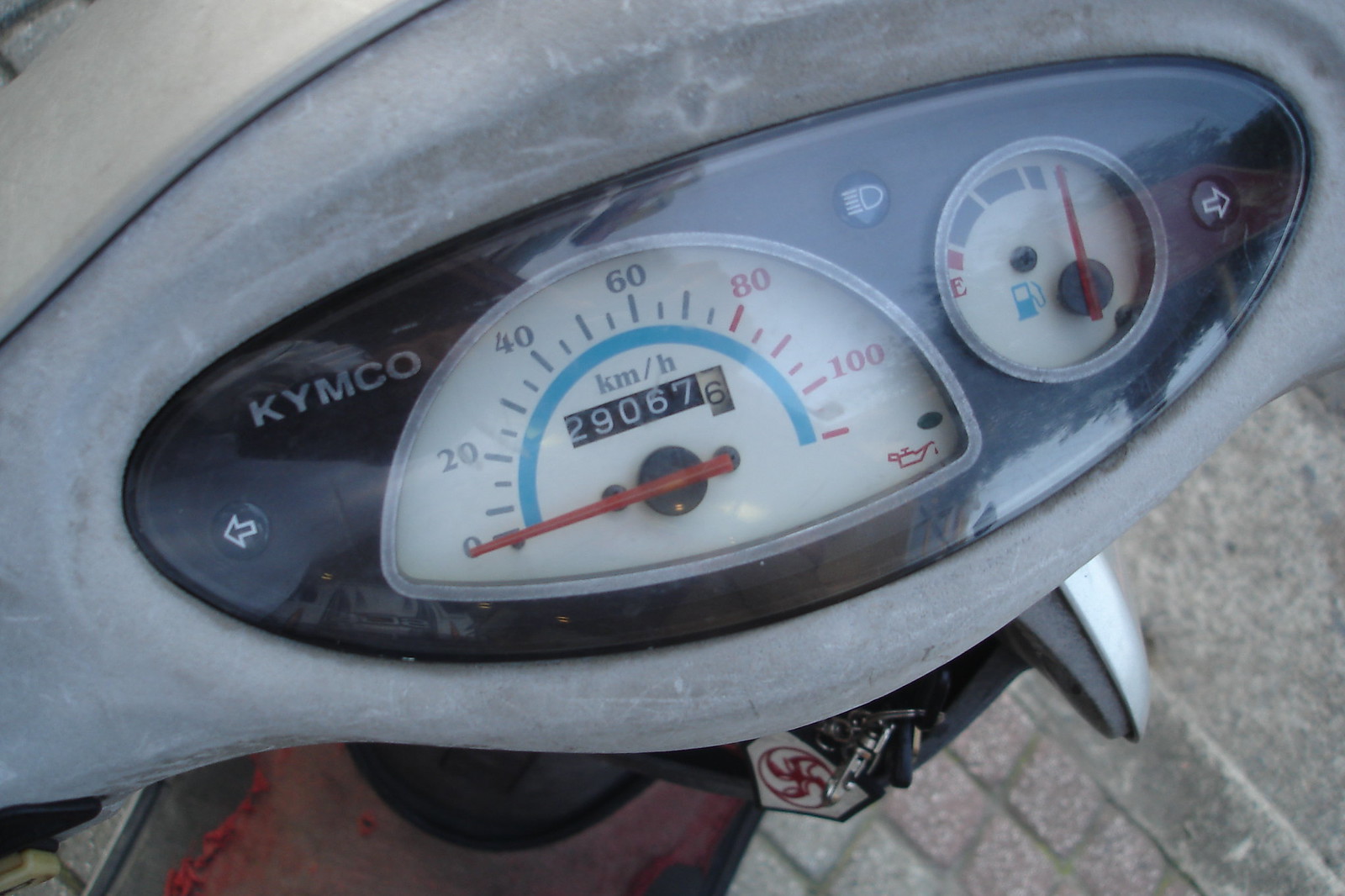The image depicts the dashboard of a Kymco-branded scooter. The central feature is a semicircular speedometer, prominently displaying the vehicle's speed in kilometers per hour, which suggests it might be a European model. The speedometer needle is pointing to zero, and the odometer shows a total mileage of 29,067.6 miles. To the right of the speedometer is the fuel gauge, which indicates a full tank. Both instruments are covered by a clear plastic shield, integrated into the handlebar assembly of the scooter. The dashboard also includes turn signal indicators, with arrows pointing left and right, and a headlight indicator. The housing surrounding the control panel is made of a faded gray plastic. Below the dashboard, a set of keys dangles from the ignition switch, hinting at the operational readiness of the scooter.